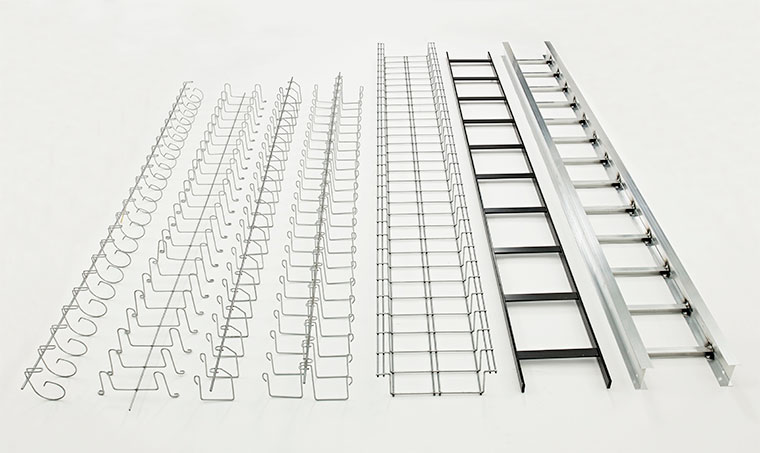The image depicts a detailed, step-by-step progression of metal structures, resembling various stages in the assembly of a ladder, displayed against a light cream-colored background. Starting from the left, the image begins with a simplistic layout featuring thin, wiry metal components, including a long vertical tube and geometric shapes akin to the letter 'G' and a broad 'M'. Proceeding to the right, the structures incrementally become more complex and recognizable as ladder parts. The configurations include what appears to be two metallic containers attached to the primary vertical tube, followed by more substantial structures similar to concrete blocks connected with handrails, mimicking the appearance of sidewalks. Continuing, the image reveals traditional ladder designs, featuring black and silver metal frames. These progressively larger and more robust ladders look as if they could support domestic tasks such as accessing a roof. Ultimately, the scene transitions from simple hangers and racks, resembling towel holders, to fully assembled ladders, portraying a fascinating evolution of design and complexity within the realm of metal structures.